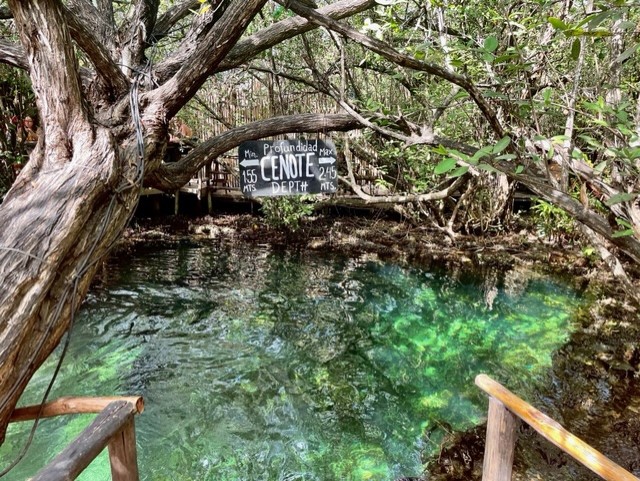This photograph reveals a serene scene deep within a heavily wooded area, showcasing a clear or greenish pond nestled in nature. The water reflects the lush green foliage that surrounds it, creating a tranquil and almost untouched atmosphere. Nearby, a simple wooden platform with primitive handrails provides an observation point for the photographer, who captures not only the water's calm surface but also a large, likely dead tree leaning over the pond.

Dominating the background of the image is a prominent black sign with white text, indicating that this site is identified as a "CENOTE". The word "PROFUNIDAD", Spanish for depth, heads the sign, followed by specifications: "MIN 1.55 MTS" on the left and "MAX 2.45 MTS" on the right, likely indicating the varying depths of the cenote. These measurements are highlighted by arrows pointing left and right, respectively. The term "DEPT #" along with numbers 155 and 216 can be seen, although their exact meaning is ambiguous.

Adding to the rich detail, the backdrop and surrounding areas flaunt thick underbrush and foliage, with a noticeable dirt and moss border around the pond, enhancing the setting's rustic and natural allure. On the far left side of the photograph, partially obscured by trees, there seems to be a glimpse of a person wearing glasses and a brown sweater, peering through the dense greenery. This detailed composition encapsulates a hidden, somewhat mystical scene in the heart of nature.